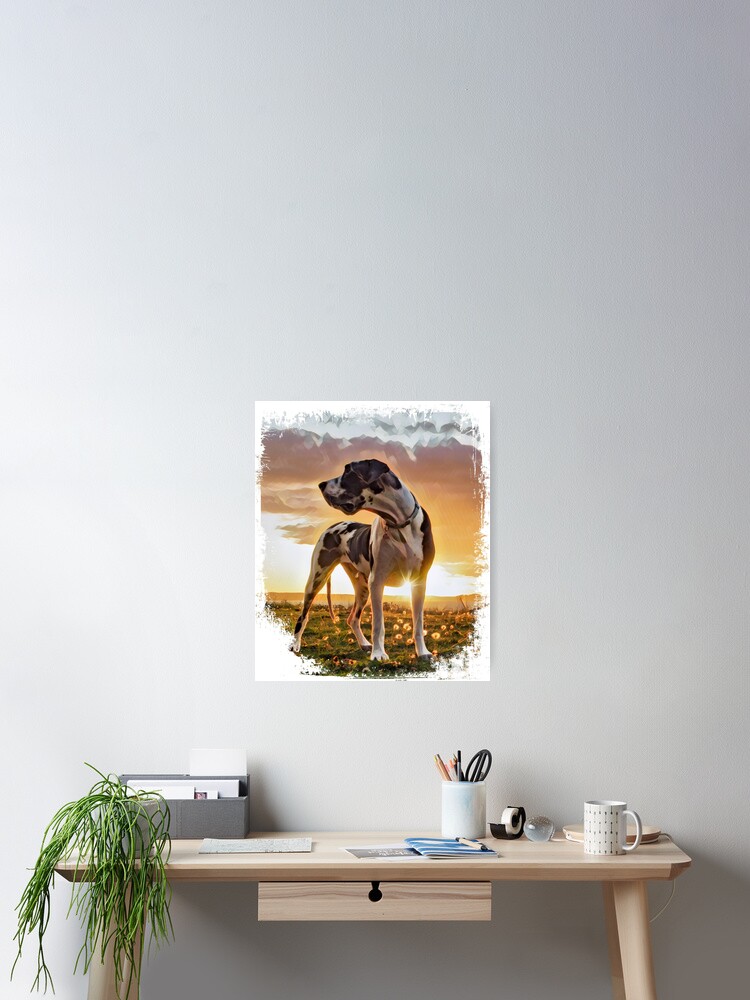The image portrays a home office setup against a very tall, white wall. The focal point is a simple rectangular desk, likely made of beechwood or light walnut, with four legs and a centered pull-out drawer. Positioned prominently on the desk are various items: on the right side, there's an adjustable white lamp with a cylindrical shade, a coffee mug, a roll of scotch tape, and a clear globe-shaped paperweight. Centrally located is a blue magazine with a paper placed to its left. A pencil holder filled with scissors, pens, and pencils also sits on the desk. On the left side, a potted plant is seen dangling gracefully off the edge, next to a gray index card holder or a small filing cabinet with its lid open. Directly above the desk, an artwork commands attention; it features a black and white dog, resembling either a Dalmatian or a Great Dane, gazing to its right. The dog is depicted standing in a grassy field with a sunset in the background, framed by a textured white border.